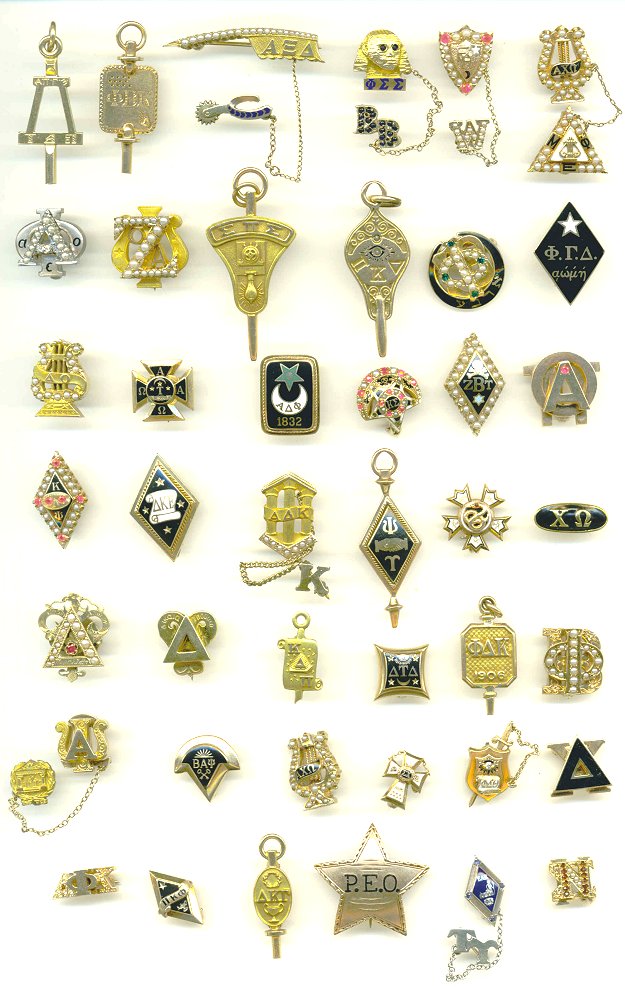This image showcases an extensive and eclectic collection of lapel pins and medals displayed against a pristine white background. The array includes both fraternity and sorority pins, as well as what appear to be notable military or police officer badges. Predominantly crafted from various metals, these pins range from gold and silver-plated to plain gray finishes, exuding a shiny and polished aesthetic.

Among the collection, several pins feature distinctive Greek letters, such as A-E-A and ZBT, suggesting affiliations with Greek organizations. Some pins are adorned with embellishments like pearls, rhinestones, and intricate engravings, adding a layer of intricate detailing. The designs vary widely: there are round pins, diamond-shaped ones, fan-shaped, shield-shaped (reminiscent of police badges), and even keychain-like designs. Notably, one pin is a pink shield with a 'W' hanging off it, while another features a prominent star with 'PEO' inscribed on it.

Additional unique elements include pins with black enamel paint, engravings of eyes, skeleton motifs, and a triangle studded with white pearls. The array boasts 6 pins across and 8 in columns, suggesting a thoughtfully organized collection of 48 distinct pieces, each carrying its own story and significance. This assortment vividly illustrates a colorful spectrum of symbols and iconography, capturing the diverse spirit of academic, professional, and possibly international cultures.